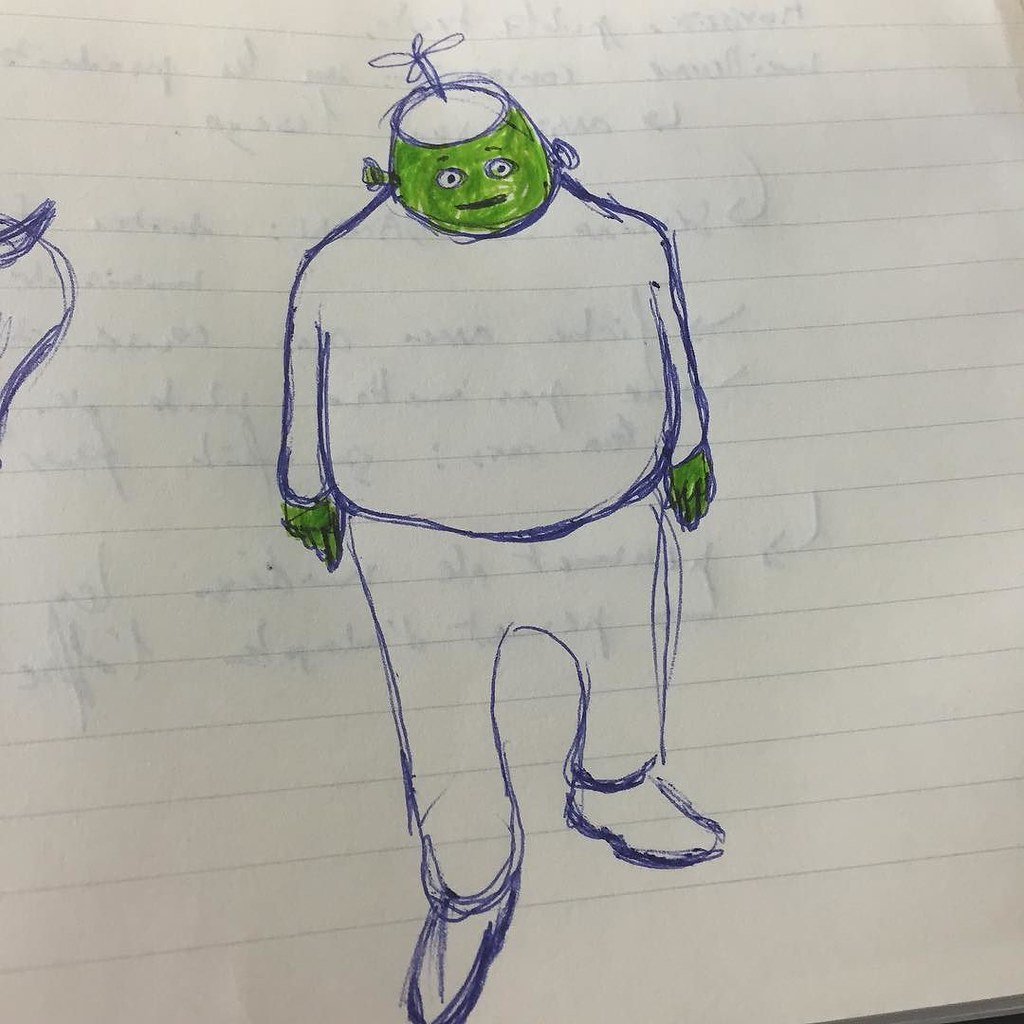In this square image, we are looking at a piece of lined paper reminiscent of what you would find in a schoolbook or loose-leaf composition book. Centered on the paper is a pen-drawn figure, meticulously outlined in blue ink. The figure features a robotic character with a human-like body, appearing chubby and dressed in pants and a long-sleeved shirt. Atop its head sits a cap, complete with a whimsical little propeller. Despite its humanoid attire, the character's green face—colorized possibly by a marker—reveals its robotic nature, highlighted by mechanical screws in place of ears. The dangling arms end in green hands, adding to its unique appearance. To the left of this main figure, there is a partial drawing, hinting at another character with a horn protruding from its head.